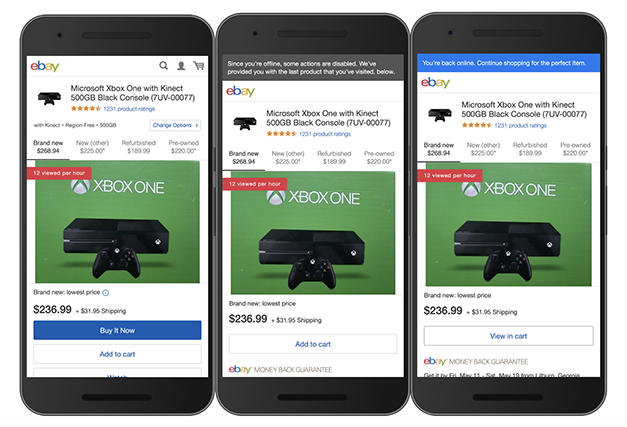This digital image features three smartphones placed side by side, each displaying listings for the same product on eBay. 

The first smartphone screen prominently shows the eBay logo and a detailed listing for a Microsoft Xbox One with Kinect, model 7UB-00077. The Xbox One, with its sleek black 500 GB console, is pictured in a large, high-resolution image. The price is clearly stated as $236.99, plus $31.95 for shipping. Below the price, there are two actionable buttons: "Buy It Now" and "Add to Cart."

The second smartphone screen displays an identical listing for the same Xbox One, replicating the price and item details. However, a message at the top reads, "Since you're offline, some actions are disabled. We've provided you with a list product that you validated below." The writing appears slightly blurry, affecting readability.

The third smartphone screen has a message indicating a change in status: "You're back online. Continue shopping for the perfect item." This message suggests that internet connectivity has been restored, allowing the user to resume their shopping activities.

The image effectively conveys the seamless integration of e-commerce on multiple devices, highlighting the continuity of the shopping experience despite network interruptions.